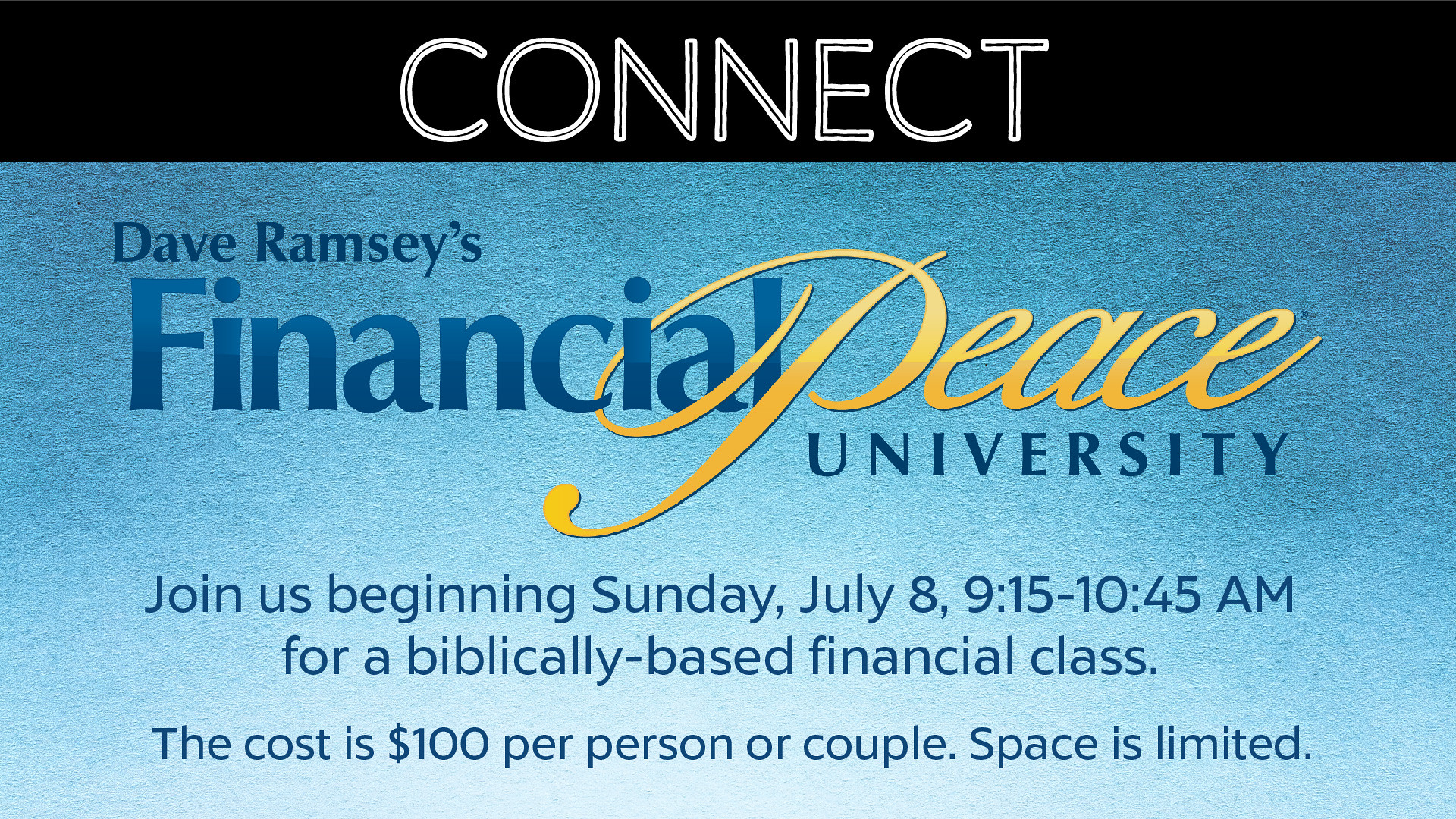The promotional image for a financial class is a landscape-oriented, rectangular ad with detailed typography and graphic design elements. At the very top, it features a thin black rectangle with the bold white text "CONNECT" centered within it. Below this, set against a gradient blue background that transitions from dark at the top to light at the bottom, is the main informational text. This text includes "Dave Ramsey's" in a dark blue font, followed by "Financial Peace University" with "Financial" in large blue letters and "Peace" in cursive gold, looping elegantly through the "I", "A", and "L" of "Financial." Beneath this, in navy blue text, it reads "JOIN US BEGINNING SUNDAY, JULY 8TH, 9:15 TO 10:45 AM" on a single line, followed by "for a biblically-based financial class." Further down, additional blue text states, "THE COST IS $100 PER PERSON OR COUPLE. SPACE IS LIMITED." The overall design uses a combination of bold, italicized, and scripted fonts to convey the information clearly and attractively.